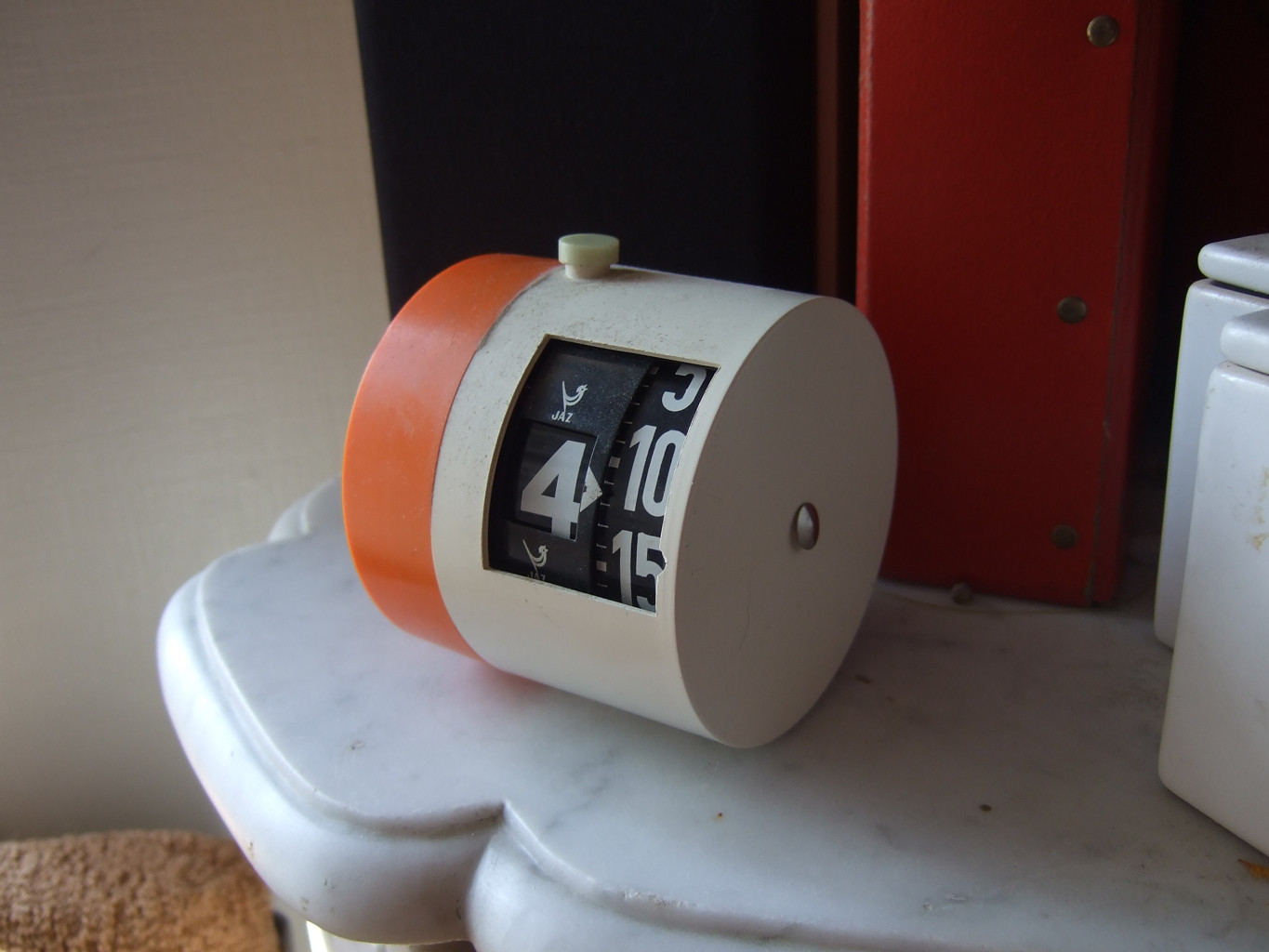The image depicts a white and gray marble-patterned surface with a cloud-like decorative appearance. On this surface, to the left, there is a red and black binder or book. In the right-hand corner, there are worn, ceramic white canisters, one of which has a lid. Centrally positioned on this surface is a distinctive cylindrical clock that resembles a barrel. This clock has an orange end and a beige body with a clear window. Inside, white numbers are displayed on a black background; notably, it points to 4 and nearly 12, suggesting an unusual clock style. A white bird emblem with the word "jazz" and a small button on top adds to its unique design. Additionally, a glimpse of brown carpet is visible at the front edge of the image.